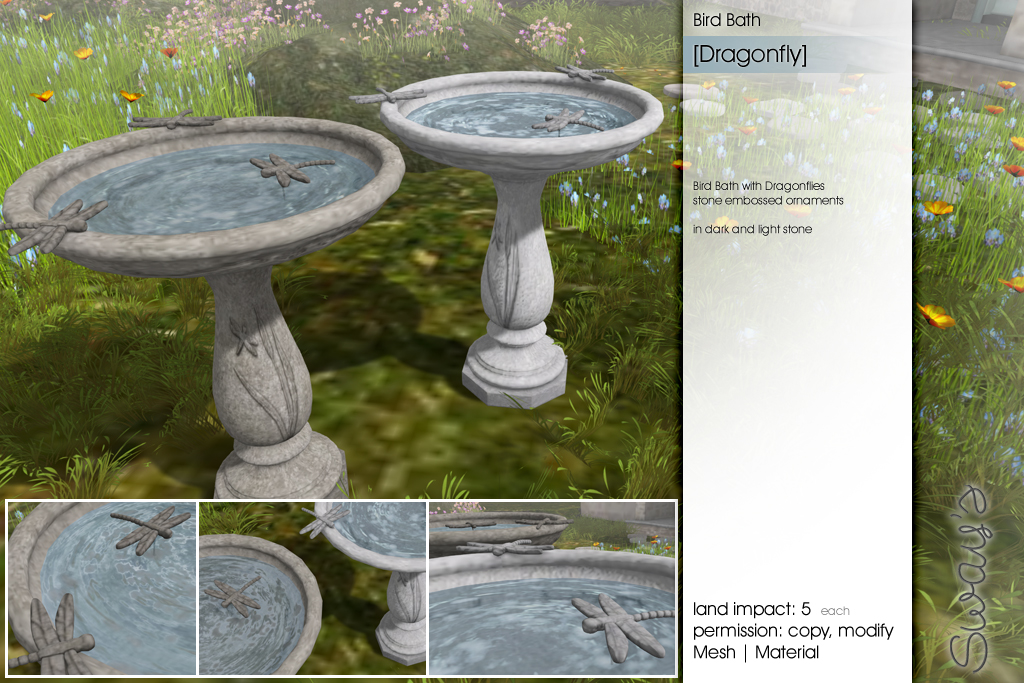This advertisement showcases two concrete birdbaths adorned with dragonfly designs, set in a picturesque country garden brimming with wildflowers. The artist's rendition vividly brings to life the scene with dark gray and almost white birdbaths, each featuring ornate dragonfly decorations both on the sides and within the shallow bowls filled with water. Surrounding the birdbaths, a vibrant array of small yellow, blue, and white flowers accentuates the tranquil outdoor setting. Along the right side of the image, a vertical white banner contains various descriptions about the birdbaths, while the artist's signature is nestled in the lower right-hand corner. At the bottom of the main image, three close-up photographs provide detailed views of the birdbaths' intricate dragonfly embellishments, enhancing the viewer's appreciation of the design.